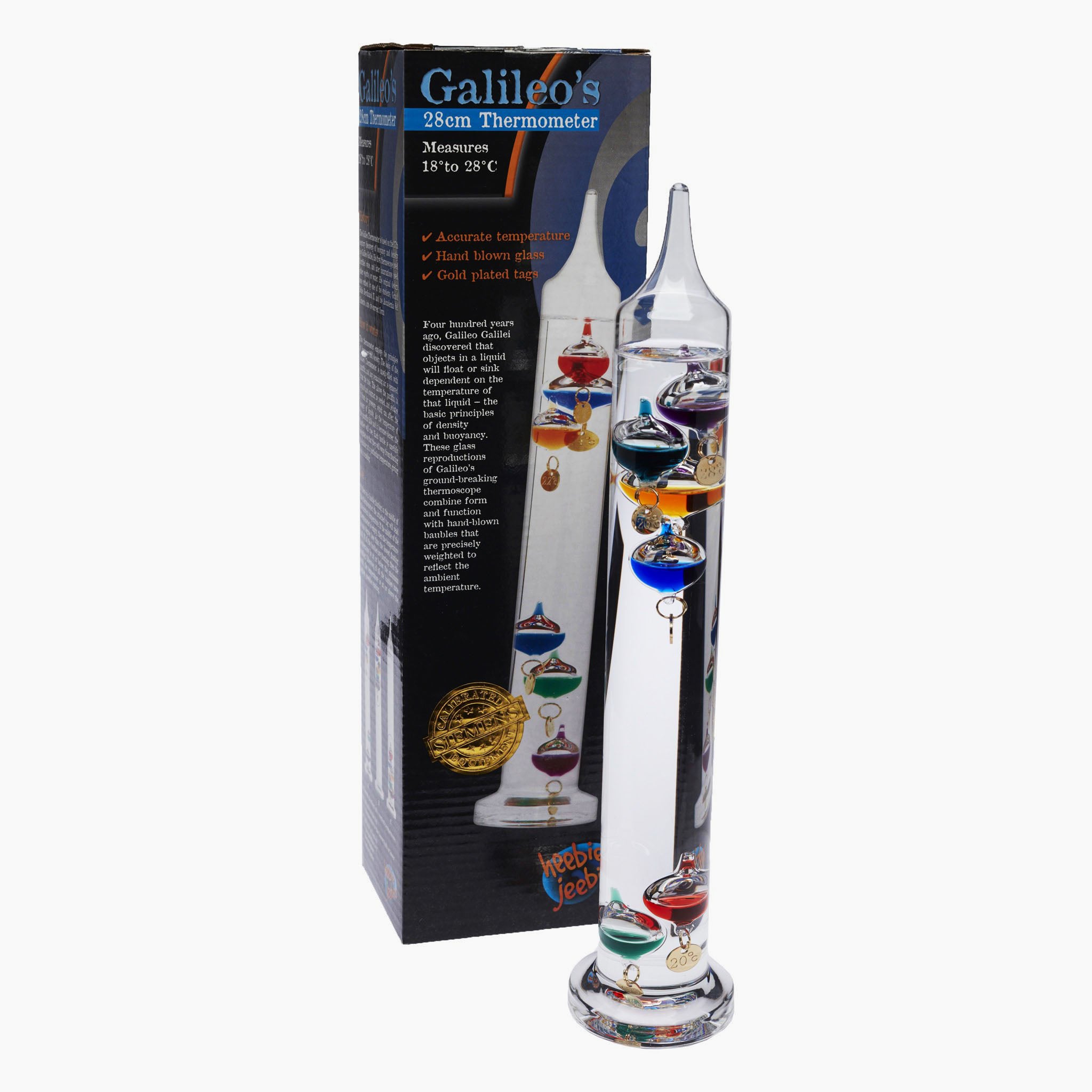The image showcases a detailed view of a Galileo thermometer and its packaging against a white background. The tall rectangular box, approximately 8 inches high, has a black upper section with light blue text reading "Galileo's 28 centimeter thermometer." Below, white text indicates it "measures 18 to 28 degrees Celsius." Further down, descriptions in orange letters highlight its accurate temperature readings, hand blown glass construction, and gold plated tags. Notably, it features check marks in brown or red next to these features. A gold seal with "Hebe Jebe" in orange letters sits at the box's lower center within a blue oval. The box's front depicts the thermometer and includes a historical note about Galileo's discovery 400 years ago regarding buoyancy and density principles—objects in liquid will float or sink depending on temperature.

The thermometer itself, which is removed from the box and placed to its right, consists chiefly of glass. Shaped like a cylinder or tube with a thick glass base, it ends in a nozzle-like top. Inside the clear glass tube, there's liquid and several colorful, spherical objects that float at different levels. These objects include purple, green, orange, blue, and red spheres, reflecting how the thermometer measures temperature.